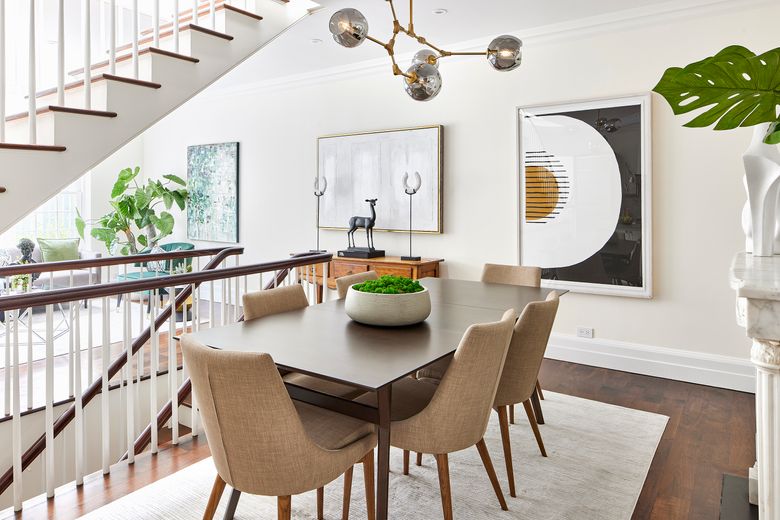This detailed image is a 3D color illustration, likely created in an app such as SketchUp, depicting the interior elevation of a modern dining room loft area. The focal point is the dining table positioned in the center with its legs over a cream-colored area rug. The table itself is dark stained wood, rectangular in shape with a low white round vase containing green foliage placed centrally. Surrounding the table are six upholstered chairs with beige tweed seats and brown legs. This setup sits on a cream area rug, which provides a soft contrast to the brown hardwood floor.

To the right side of the room, there's a partial view of a white fireplace mantle adorned with a modern vase holding a large green leaf. On the walls, several framed pieces of art are displayed, including a modern art poster featuring a white semicircle with accompanying black and orange elements and black lines. Nearby, there are two additional framed portraits in green and blue hues with floral motifs.

Prominently featured on the left side is a stairwell that ascends to and from the dining loft area. This staircase showcases a white picket and dark wood handrail with the horizontal railing also brown on top, giving it a grid-like appearance. Above the table is a distinctive chandelier fixture that resembles antlers, made from brown brass and adorned with round silver globes.

The overall ambiance of the room is bright, illuminated by natural daylight. The modern and airy feel is accentuated by the presence of a standalone pot with a ficus tree, and a side table displays an iron deer sculpture and horseshoes mounted on metal posts. This room is designed to reflect a blend of contemporary and rustic styles, capturing an inviting, lived-in aesthetic.